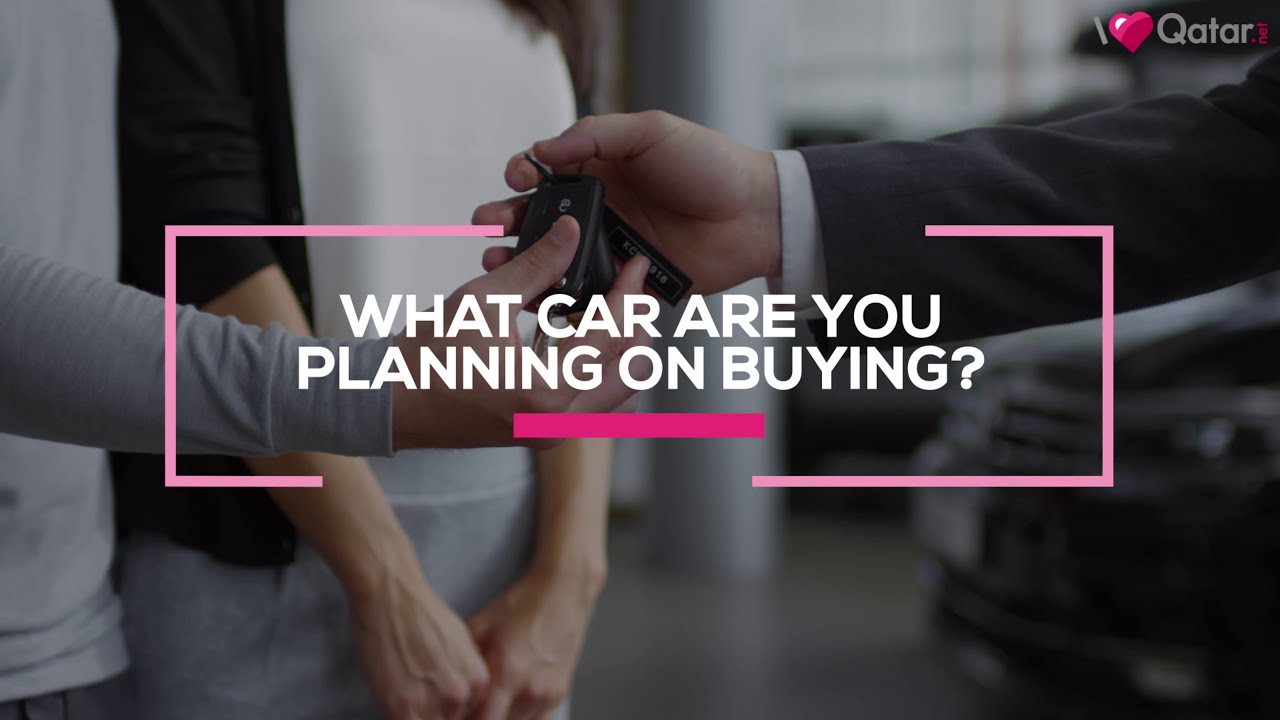The image is a graphic advertisement set in a car dealership showroom. The background features a slightly grayed-out photograph of a man and a woman accepting car keys from a salesman. The man, who is wearing a gray long-sleeved t-shirt, is receiving the keys from a salesman dressed in a suit with a white shirt. The woman next to him, dressed in a white blouse, black sweater, and gray skirt, has her hands clasped in front of her. The scene captures the moment with a blurred car visible in the showroom behind them and a round, gray pillar rising in the middle. Superimposed on the image, in the center, is the text "What car are you planning on buying?" in white capital letters with bright pink borders and a dark pink underline. In the upper right-hand corner, there's a logo that says "I ♥ Qatar," with 'I' and 'Qatar' in gray text and the heart symbol in pink.